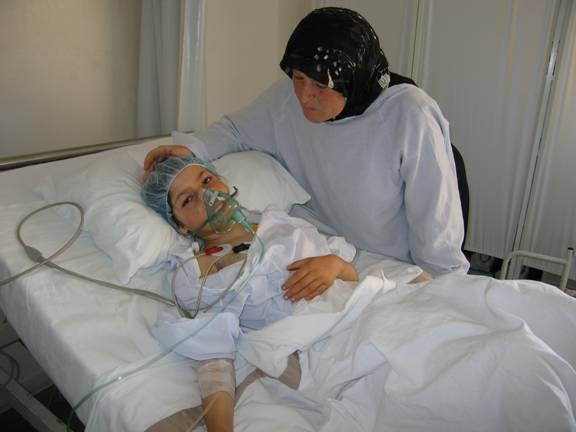In this poignant photograph set in a medical facility, a young white girl lies in a hospital bed covered with white sheets pulled up to her chest. She wears a light blue hospital gown and a blue surgical hairnet on her head. An oxygen mask, light green in color, rests over her face with cords trailing down her shoulders and over the bed. Her right hand is placed gently on her stomach, while her left arm lies to her side, secured with an IV. Monitors are visibly attached to her chest, indicating her critical condition. Leaning over her with a caring and protective demeanor is an older white woman, adorned in a white hospital gown that drapes over her front. She tenderly places her right hand on the girl's head, her expression emanating concern and affection. The woman wears a black scarf that gracefully wraps around her head and extends down her back, further highlighting the intimate and compassionate nature of the scene.